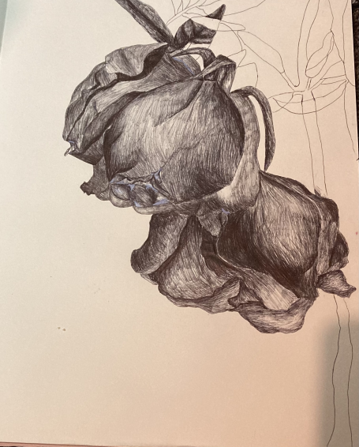This image depicts a detailed pencil drawing of a partially complete flower on a white background. The main subject appears to be a plant with two prominent flower bulbs, one partially open and the other closed, resembling blooms hanging upside down from a stem. The shaded areas are executed in black and gray pencil with an intricate touch that adds depth, and there is a very light touch of blue in the middle of the partially open flower. The petals, which have a flowing, romantic quality akin to billowing skirts, contribute to an evocative and dreamy atmosphere. In contrast, the right side of the image remains unfinished, featuring simple line drawings of stems and leaves without shading, adding to the sense of an ongoing work-in-progress. The background includes additional outlined foliage, enhancing the layered composition of the drawing.